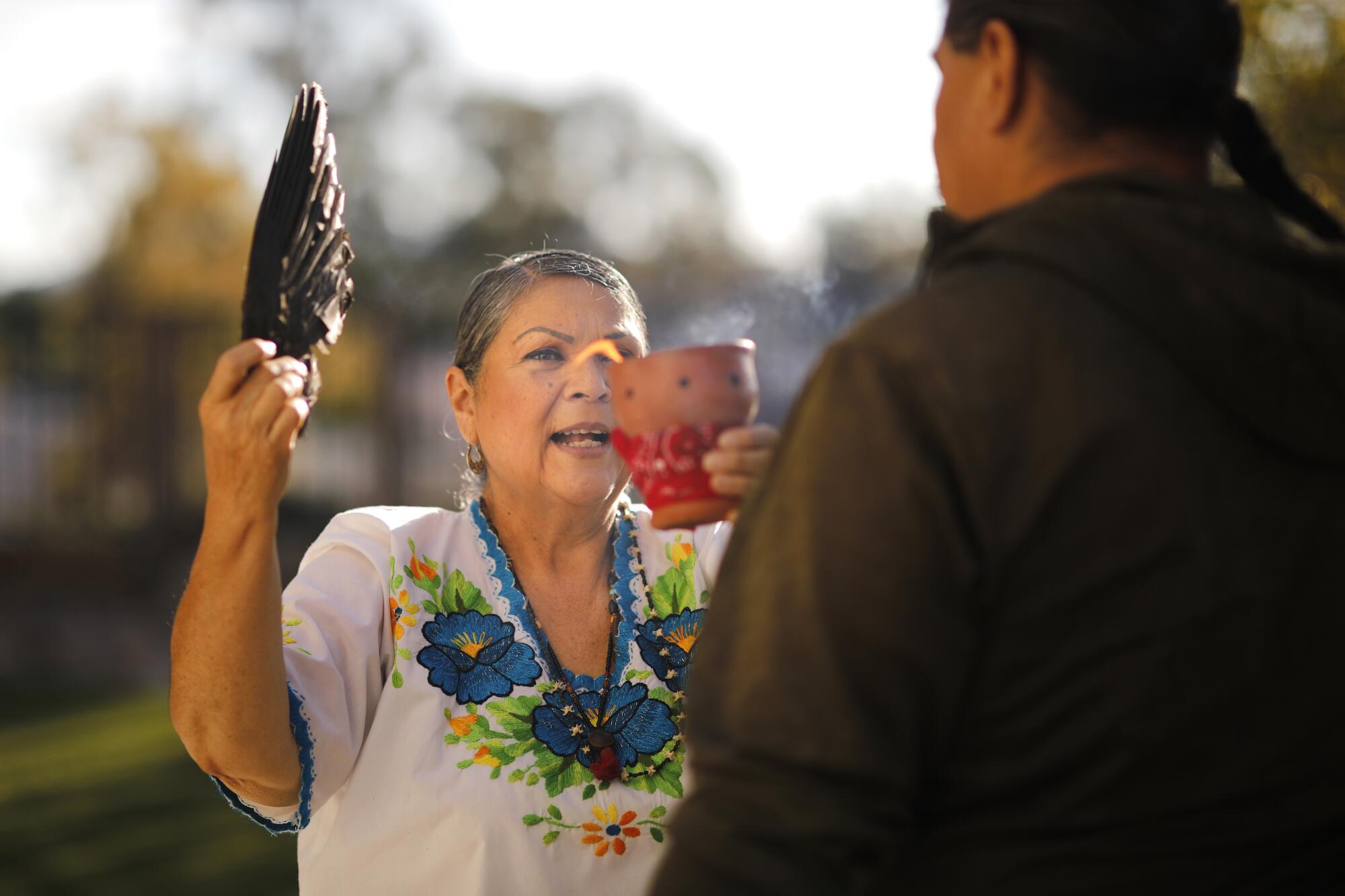In this outdoor, daytime photograph, an older woman stands on the left side, facing a man on the right whose back is towards the camera. The man, characterized by his long, braided ponytail and dressed in a dark, long-sleeved shirt or jacket, appears to be attentively listening to the woman. He stands with only his back visible, allowing a clear view of the woman.

The woman, in a short-sleeved, white V-neck shirt adorned with a blue floral pattern and green leaves, holds a clay pot with red patterns in her left hand. Smoke is emanating from the pot, suggesting it might be burning something inside. In her right hand, she holds a large black feather, possibly a bird's wing, using it like a fan. Her focus is on the man, holding both items near eye level as if presenting them to him.

The background is very blurry, displaying a white sky, some indistinct trees, and possibly a body of water, enhancing the serene and somewhat ceremonial tone of the image.